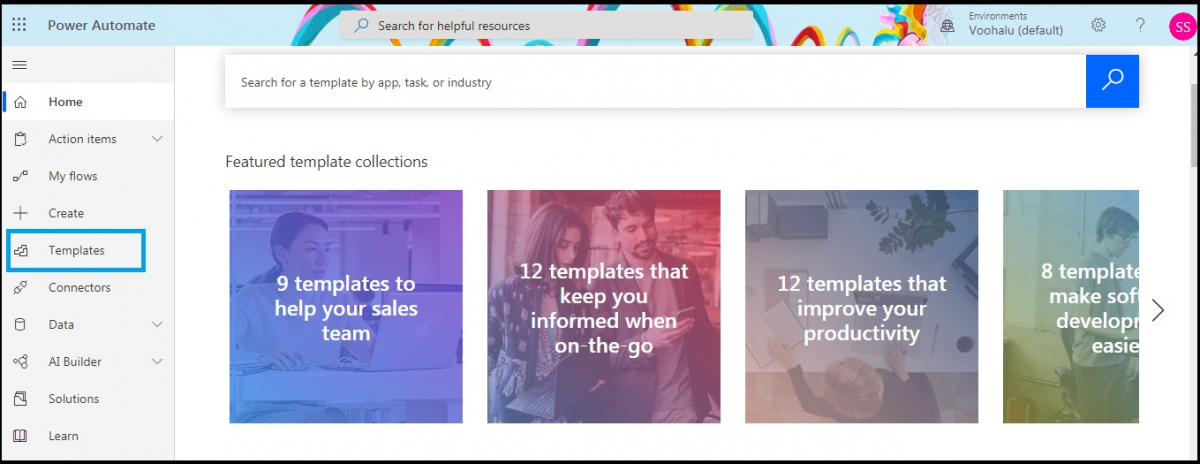The image showcases an interface, likely from an application or a website, primarily utilizing a white background with black text. At the top of the page, there is a light blue bar adorned with a rainbow-colored theme. This bar features the text "Power Automate," along with a gray search box labeled "Search for Helpful Resources." On the right end of this bar, the segment displays "Environments," "Vuhalu," "Default," alongside icons for settings (gear), help (question mark), and a pink circle with the initials "SS" indicating a user profile icon.

To the left of the page, a vertical gray pane lists several navigation options: "Home," "Action Items," "My Flows," "Create" (with a blue rectangle highlighting it), "Templates," "Connectors," "Data," "AI Builder," "Solutions," and "Learn."

The main section of the page contains a prominent search box labeled "Search for Template by App, Task, or Industry" accompanied by a blue magnifying glass button for initiating the search. Below this, a section titled "Featured Template Collections" is displayed, featuring various images with corresponding text:

1. An image of a woman with the caption "9 Templates to help your sales team."
2. An image of a woman and a man with the caption "12 Templates that keep you informed when on the go."
3. An image of a woman at a desk with the caption "12 Templates that improve your productivity."
4. An image of a young man with the caption "8 Templates that make software developing easy."